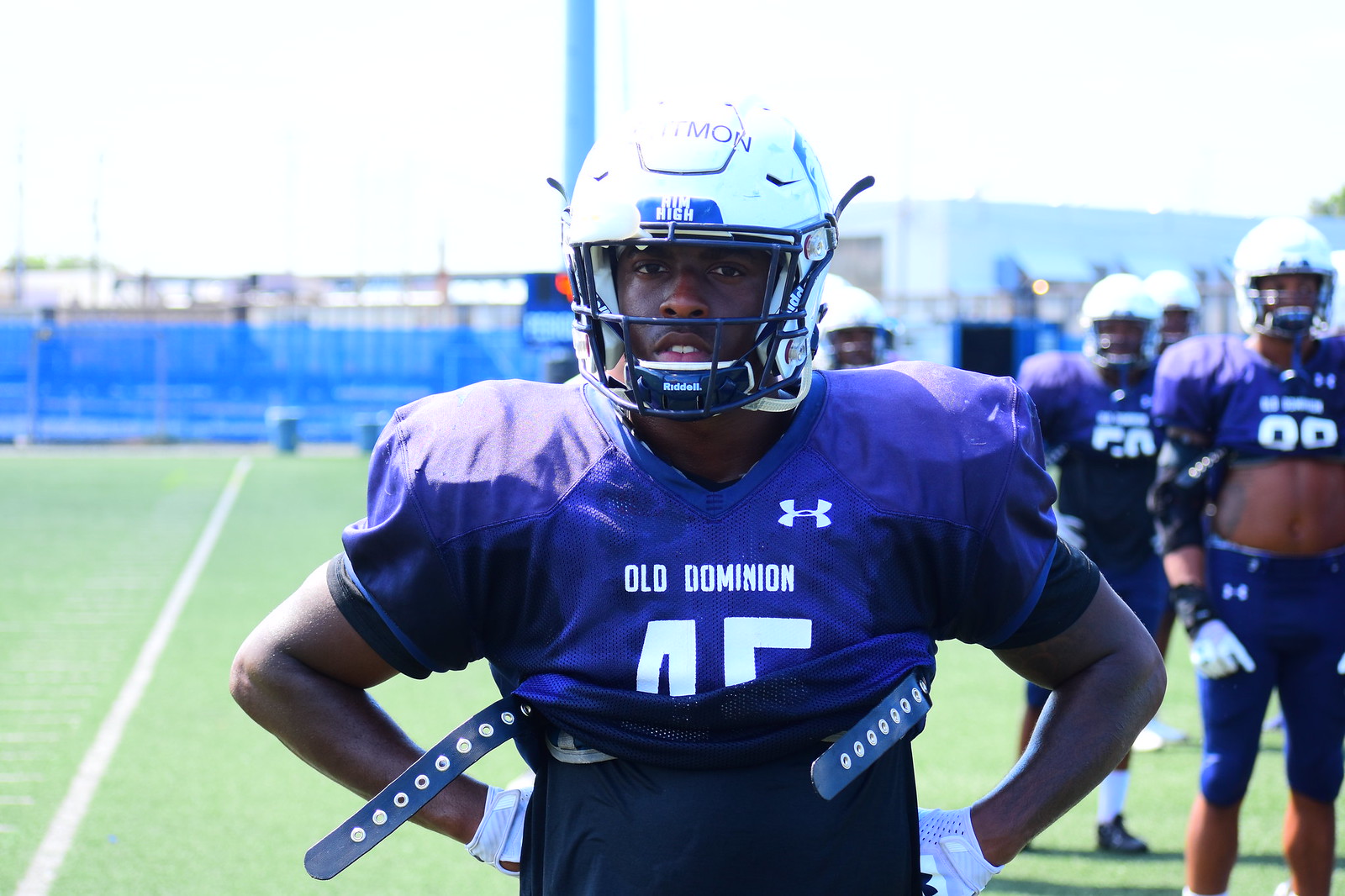The image captures a close-up shot of a college football player from Old Dominion University, standing on a lush green football field with white yardage lines visible. The focal point is an African-American player wearing a purple jersey with the number 45 and the words "Old Dominion" alongside an Under Armour logo on the chest. He is equipped with a white helmet and white gloves, and his jersey is pulled up to his midsection as he stands with his hands on his hips. More players wearing identical purple jerseys and white helmets can be seen in the background, though they are out of focus. To his left and right, teammates can be observed, one with the number 99 and another with the number 50. The stadium edge, featuring blue bleachers, is faintly visible in the background.